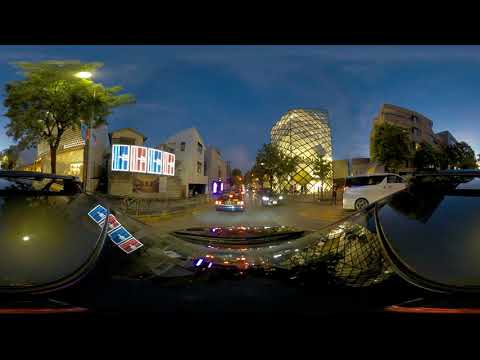This detailed photograph captures a night scene in an urban, upscale neighborhood, seemingly taken from the dashboard of a vehicle. The image is slightly distorted, possibly due to a panoramic or wide-angle lens. Dominating the center of the frame is a two-lane road with multiple cars approaching, their headlights casting reflections on the shiny black hood of the vehicle from which the photo is taken. The ambient twilight blue sky indicates that the time is around dusk or early evening. 

On the right side of the image, a white SUV is parked, and further in the background, a sophisticated, tall, square-shaped glass building glows with intricate, backlit patterns, contributing to the area's posh atmosphere. Adjacent to this building are additional structures, including a modern two-story building and a red-blue lit signboard. 

On the left side of the street, various buildings range from two to four stories high, one of which features a peaked roof. Prominently displayed is a theater or marquee with a well-lit, rectangular sign. In the foreground, a potential traffic circle is discernible, adding to the dynamic urban layout. Trees and a street lamp are visible in the background, adding a touch of greenery to the scene. The entire area is bathed in artificial lighting, enhancing the street's premium and well-maintained appearance.